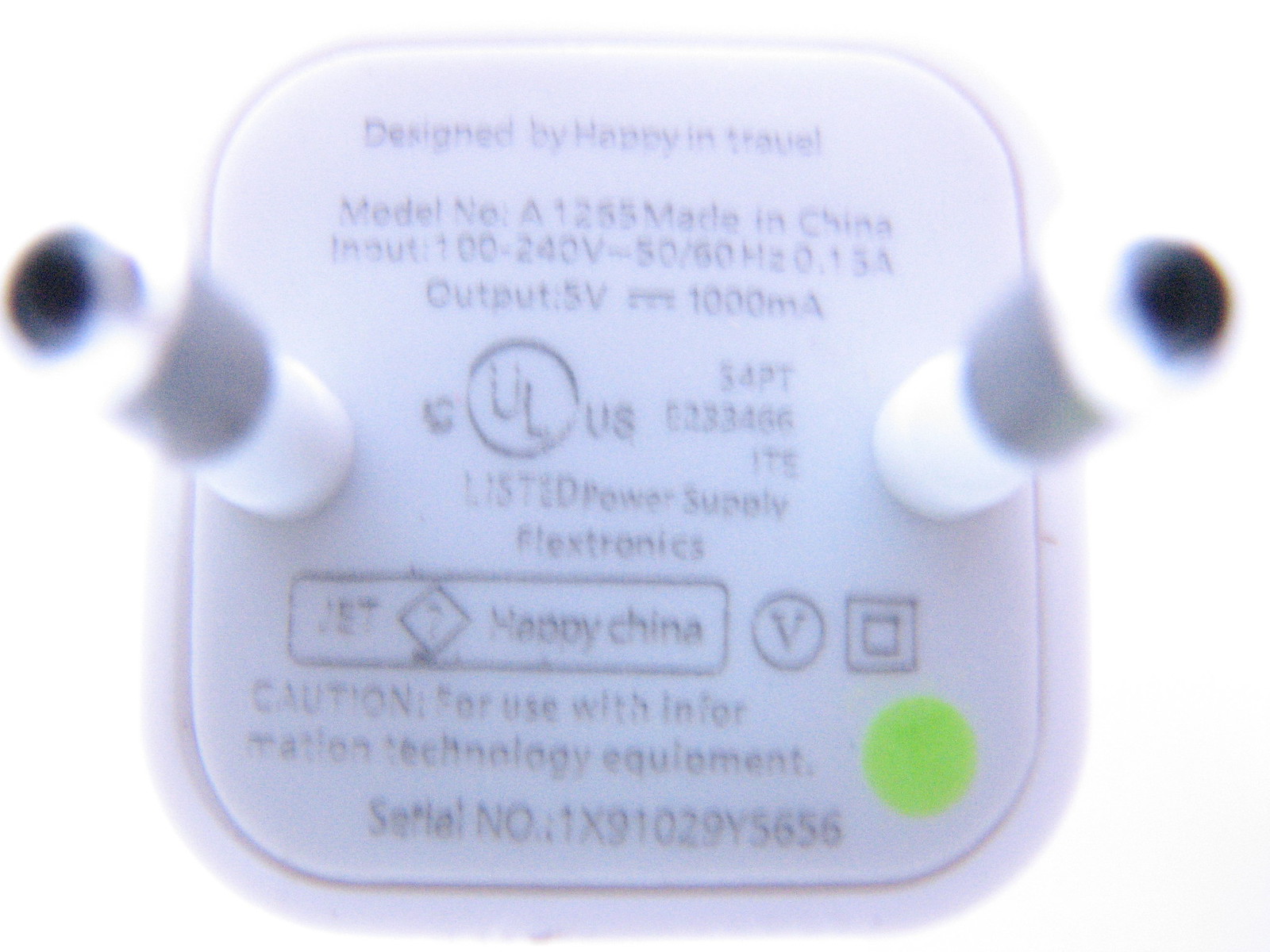This photograph captures an electronic device against a stark, plain white background. The object, slightly blurry and out of focus, has a square shape with rounded edges. Two cylinder-shaped, antenna-like protrusions extend from it, appearing as if they might plug into something. Detailed text on the device includes: "Designed by Happy in Travel," "Model Number A1255," "Made in China," "Input: 100-240V, 50-60Hz, 0.15A," "Output: 5V, 1000mA." Additionally, various symbols and markings are present: a "UL" inside a circle, a "V" inside another circle, a square within a square, a caution note stating, "Caution for Use with Information Technology Equipment," and a serial number, "1X91029Y5656." Also notable is a lime green circle positioned on the right-hand side of the device.